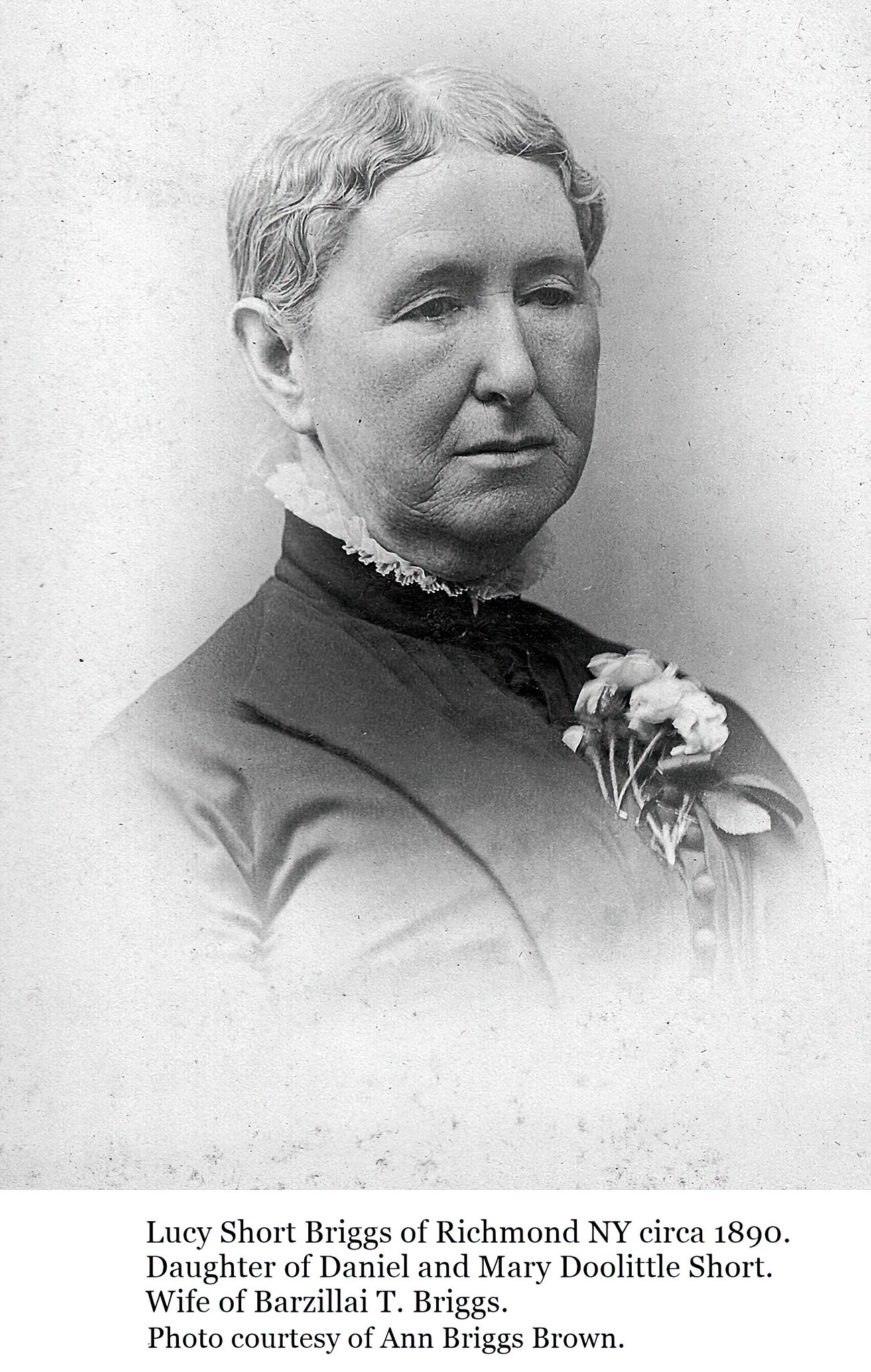This black-and-white portrait, dating circa 1890, features Lucy Short Briggs of Richmond, New York. Daughter of Daniel and Mary Doolittle Short and wife of Barzilai T. Briggs, Lucy is depicted with short, gray hair and light skin, displaying some wrinkling, indicating she is older. She appears somewhat sullen as she gazes down and to the right. Lucy is dressed in a dark coat or dress adorned with a white ruffled collar that reaches up to her neck, and she has flowers pinned to her clothing, featuring prominent leaves and white blossoms. The background is light gray, and the image fades out towards the bottom. The caption beneath the photo reads: "Lucy Short Briggs of Richmond, NY, circa 1890. Daughter of Daniel and Mary Doolittle Short. Wife of Barzilai T. Briggs. Photo courtesy of Anne Briggs Brown."